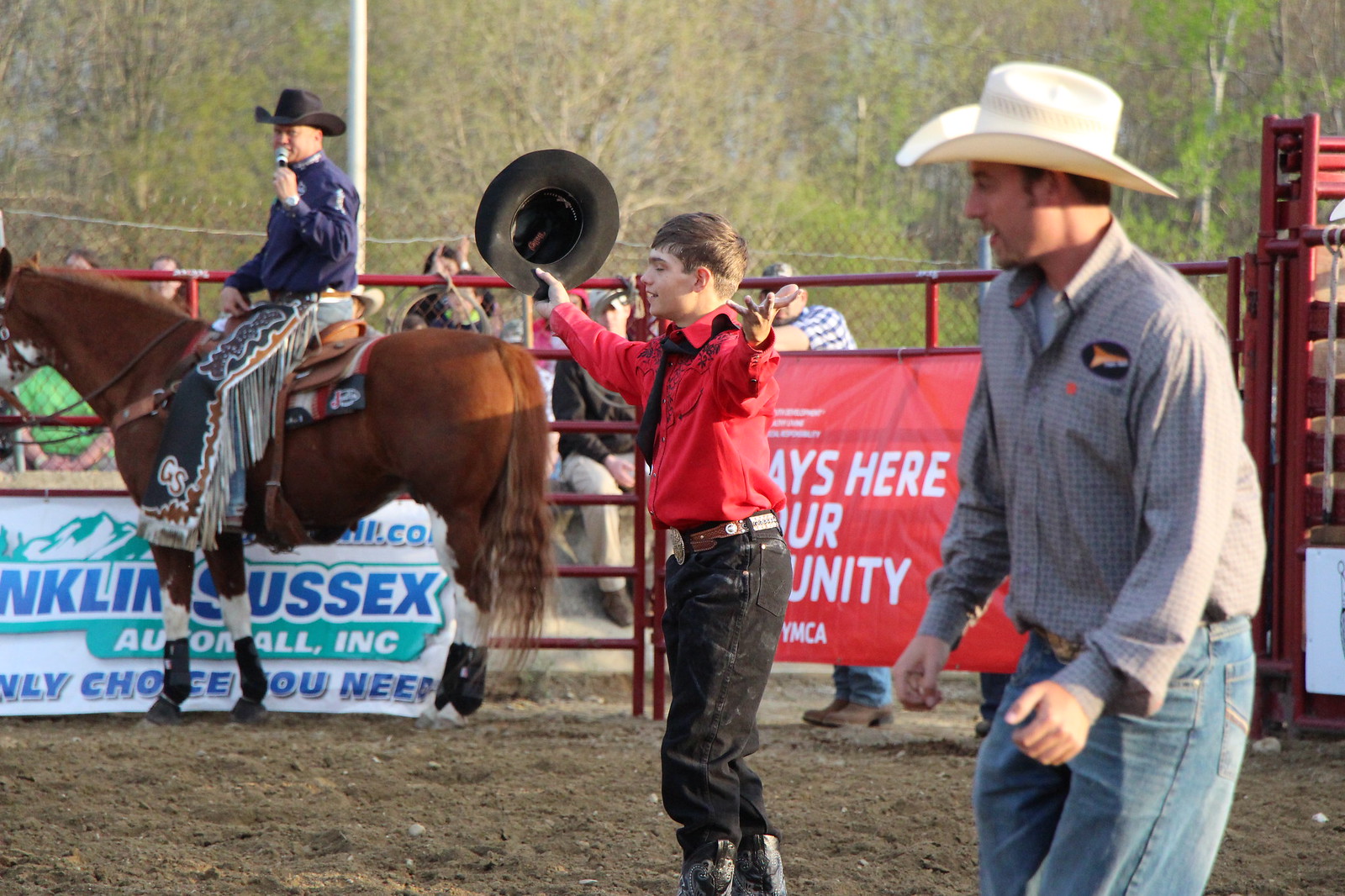This photograph captures a vibrant scene at what appears to be a rodeo, featuring three distinct figures against a bustling backdrop. On the left-hand side, a man is seated on a brown horse, holding a microphone in his left hand. He wears a blue shirt, black chaps adorned with tassels, and a black cowboy hat. His role suggests he might be the announcer or host of the event. In the center stands a boy, likely between seven and ten years old, dressed in a detailed red cowboy shirt with black ornamental stitching, black pants, cowboy boots, and a black tie. His brown hair is visible, and he holds a black cowboy hat in his outstretched right hand, as if acknowledging the crowd or taking a bow. His posture, with arms wide and eyes closed, suggests he could be receiving applause or recognition. To the right, another man stands wearing a white cowboy hat, a gray striped button-down shirt, jeans, and a belt with a large buckle. He appears to be gazing towards the boy, possibly sharing in the moment of acknowledgment. The entire scene is set on a dirt field, encircled by a red metal fence adorned with various banners, including one for the YMCA in white letters on a red background. Behind the fence, spectators can be seen sitting on benches or stands. The background also features foliage, with trees and poles visible, and a hint of blue sky peeks through the branches.